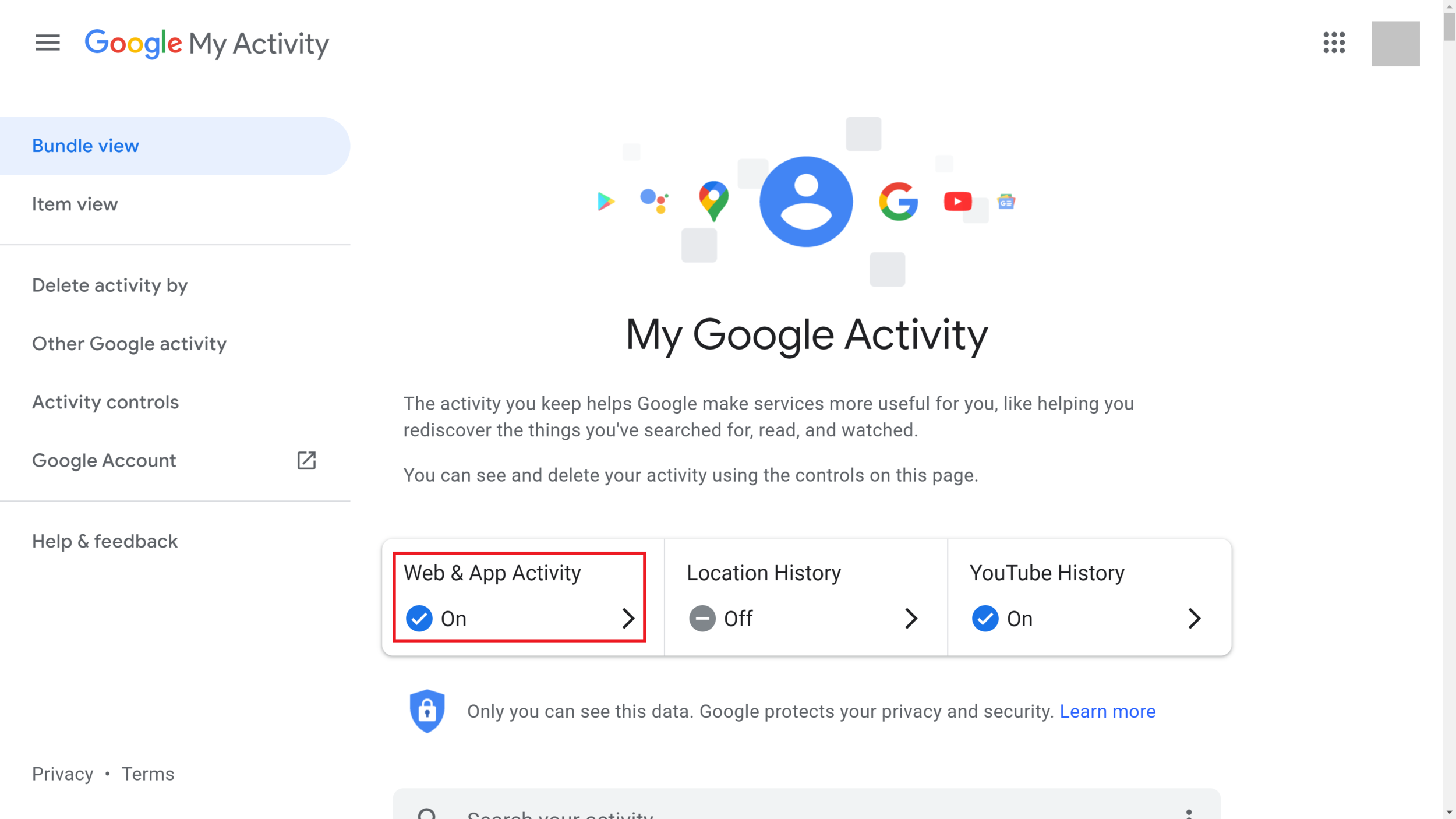Caption:

In this detailed screenshot from the Google My Activity page, the left-hand column features several navigational options. At the top, users can choose between 'Bundle View' or 'Item View.' Following a blue separator line, the options 'Delete Activity by,' 'Other Google Activity,' 'Activity Controls,' and 'Google Accounts' are listed, with an icon resembling an arrow contained in a box next to them. Beneath another blue line, links for 'Help' and 'Feedback' are available, and at the very bottom, 'Privacy' and 'Terms' buttons are visible.

On the right side of the screen is the main activity display, starting with a head-and-shoulders icon indicating the user's profile. The screen also features various icons such as a location button, a 'G' icon possibly for accessing Gmail, a red play button likely for YouTube, and another icon resembling a trash bin. Prominently, the title 'My Google Activity' is written in large, black, mixed-case letters. Below this, a statement in dark blue text explains, 'The activity you keep helps Google make services more useful for you, like helping you rediscover the things you've searched for, read, and watched.' Another line notes, 'You can see and delete your activity using the controls on this page.'

Highlighted sections indicate the status of different activity settings: 'Web and App Activity' appears as 'On' with a blue circle and white checkmark, 'Location History' is marked 'Off' with a gray circle and white line through it, and 'YouTube History' is 'On,' also with a blue circle and white checkmark. A locked icon symbolizing security notes, 'Only you can see this data. Google protects your privacy and security,' followed by a clickable blue section labeled 'Learn More.'